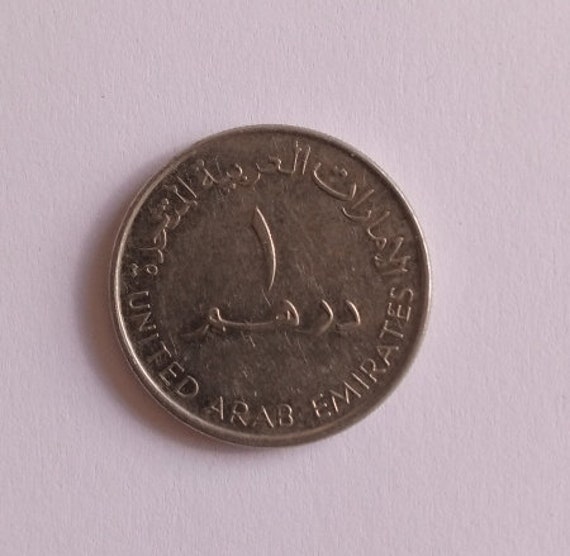This detailed photograph showcases a small coin resting on a lilac-colored background. The coin, copper or bronze in appearance with slight tarnish, features smooth edges without ridges. At the top of the coin, there is an inscription in Arabic script, while the English words "United Arab Emirates" curve around the bottom. The center of the coin displays a unique symbol or Arabic character in relief. This image focuses solely on the coin, with no other elements such as people, animals, or structures present. The coin appears to be slightly larger than an American quarter but smaller than a half dollar, indicative of currency from the UAE.